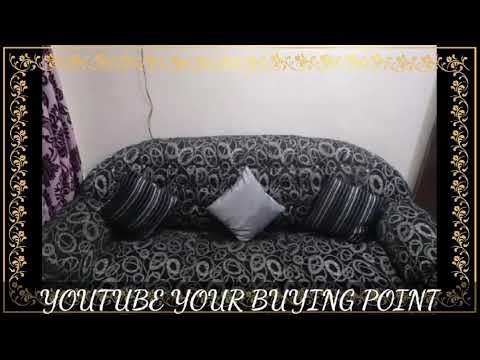This black and white image showcases a stylish black fabric couch with a rounded back, set against a gray wall. The couch, featuring a busy design of intermeshed gray circles, is adorned with three pillows: two black pillows with silver stripes on the left and right, and a solid silver throw pillow in the center, oriented like a diamond. The room has a touch of color with patterned purple curtains to the left. A black wire dangles down from behind the sofa, adding a casual element to the scene. The image is framed with an ornate floral gold trim, bordered further by a simple black line. At the bottom of the image, in white cursive font, it reads "YouTube your buying point," hinting at a possible advertisement.